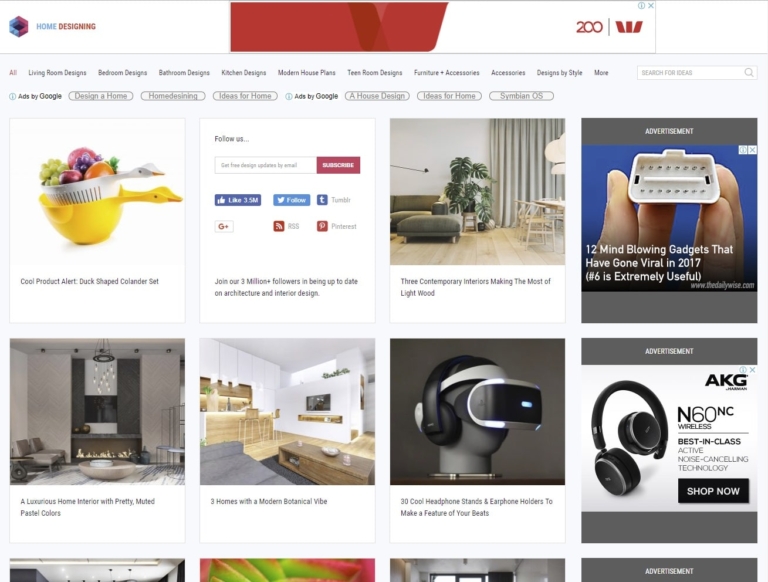This collage features several home design elements sourced from the website HomeDesigning. On the left, a "cool product alert" showcases a charming duck-shaped colander set. The set consists of a yellow and a white plastic colander, stacked together, with the white colander containing an assortment of fresh fruits including grapes, apples, oranges, and a pomegranate.

To the right, there is a vibrant image of an indoor plant, positioned in a room with beautiful hardwood floors. Adjacent is a sleek gray couch. The room exudes a contemporary vibe, enhanced further by the caption “12 mind-blowing gadgets that have gone viral in 2017,” accompanied by fingers holding a small plastic object.

Finally, another image captures the inside of a luxurious home decorated in muted pastel colors. This space features elegant lighting and a cozy fireplace, creating an inviting and sophisticated ambiance.